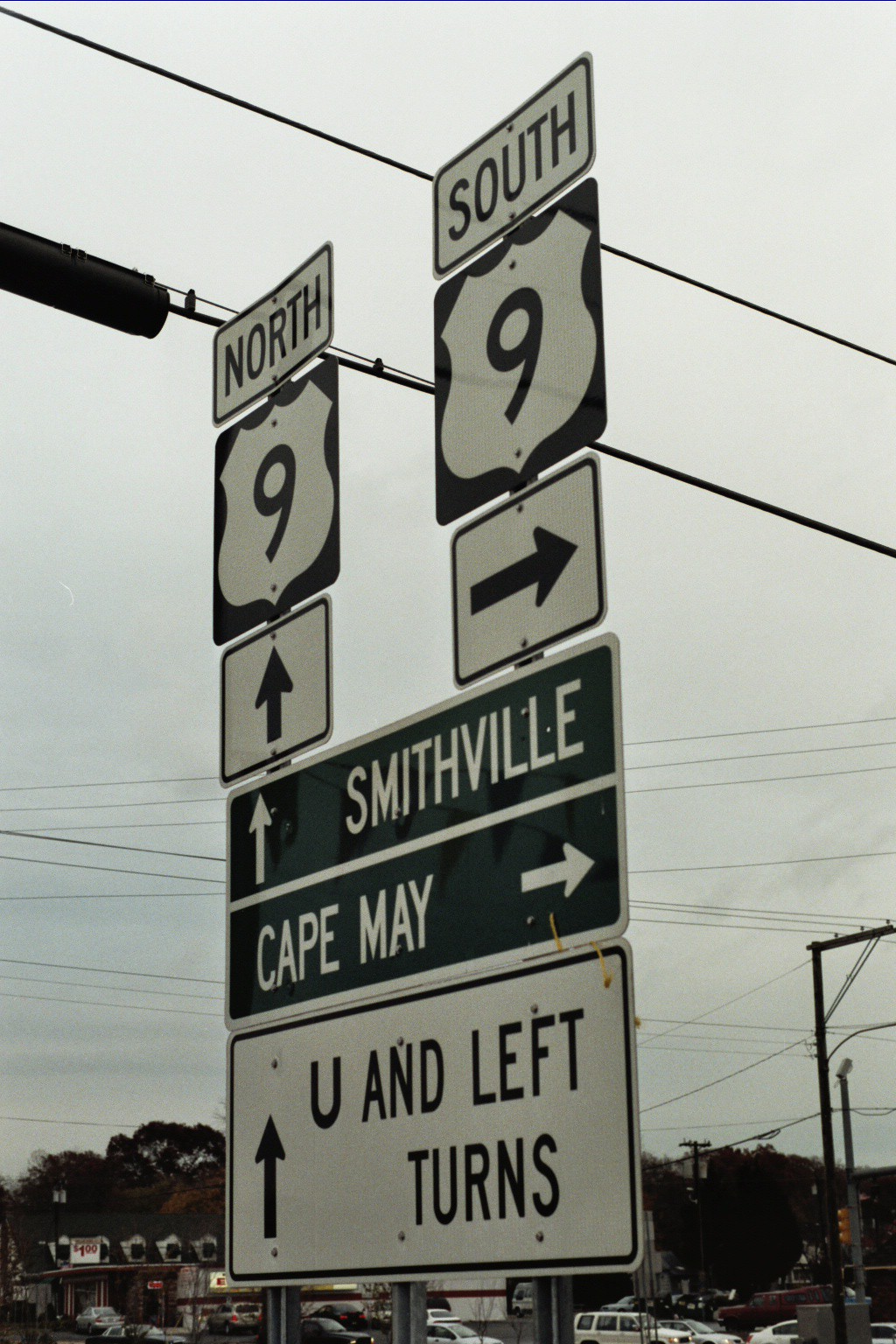The image showcases a collection of street signs at a busy intersection. Prominently displayed are signs indicating directions for Route 9, with one sign pointing north with an upward arrow, and another pointing south with a rightward arrow. Directly below, green signs with white text and arrows provide directions to Smithville (upward arrow) and Cape May (rightward arrow). Additionally, there is a sign with a white background and black text indicating the directions for U-turns and left turns with an upward arrow. The setting appears to be a bustling road, with a visible establishment that looks like a restaurant in the backdrop, its parking lot noticeably filled with vehicles. The scene is further detailed with power lines, street poles, and potentially multiple security cameras nearby.